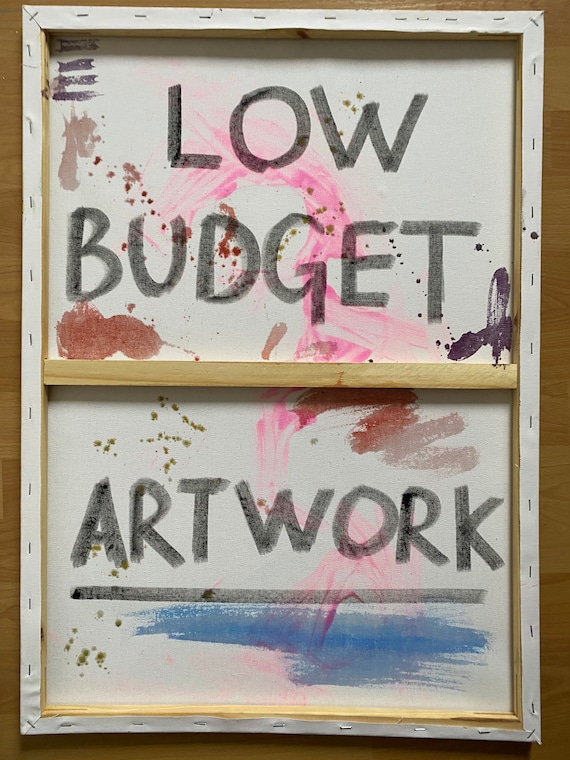The photograph depicts a vertical portrait-style canvas mounted on a wooden frame. The frame itself includes a central cross beam, giving it the appearance of a window with two panes but without glass. The canvas is loosely stapled to the wooden frame with visibly haphazard and messy staples, adding to its "low budget" aesthetic. The words "LOW BUDGET ARTWORK" are written in large black marker; "LOW BUDGET" appears on the upper pane, while "ARTWORK" is on the lower pane, underlined for emphasis. Surrounding the text are various smudges and streaks of paint in blue, pink, red, green, and purple, which seem randomly applied, further reinforcing the theme. The cross beam and unpainted wood contribute to the overall makeshift look. The piece appears to be satirical, playing on minimalist and ironic art concepts.